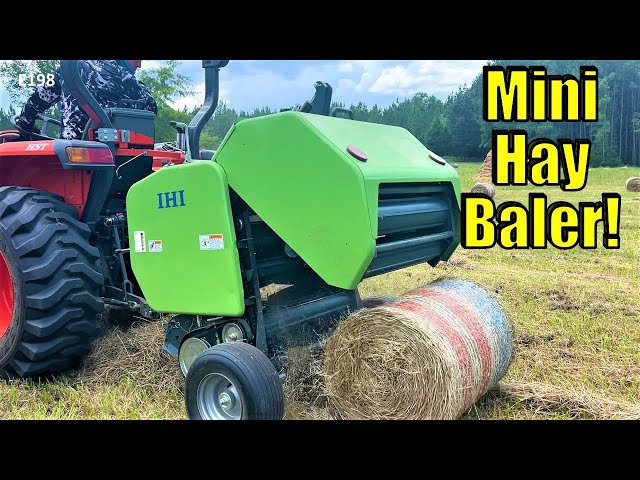The photograph showcases a vividly colored green and red mini hay baler in a sunlit field of vibrant green grass. The vehicle, equipped with wide, black tires, is actively rolling hay into barrel-like shapes and securing them tightly with string. The machine has distinct red parts at the front and green at the back. The scene is accentuated by a thick black border on the top and bottom of the image. A yellow text with a black shadow reading "mini hay baler" is prominently displayed in the top right corner. There is also an "E198" and "IHI" label on the hay baler. A man sits on a small red tractor attached to the hay baler, driving it across the field. In the background, several completed hay bales dot the landscape, and a wooded area with large trees frames the horizon. The sky above is bright blue, speckled with fluffy white clouds, adding to the serene rural ambiance of the scene.